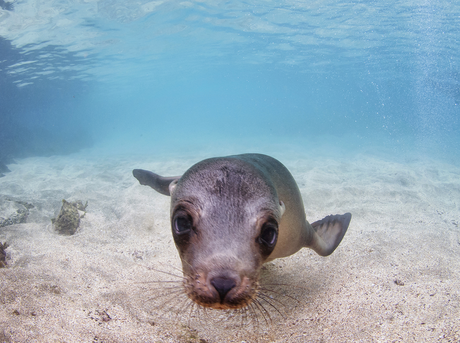In this underwater photograph, a gray seal is centrally positioned near the bottom of the frame, floating just above a sandy, pebble-strewn seabed. The seal's large, whiskered face is prominently featured as it looks directly into the camera with a curious yet somewhat sleepy expression. Its body stretches back, tapering towards the right, with two visible fins extending from its sides. The scene is bathed in the deep blue hues of clear water, with the surface faintly visible above. The setting captures the serene simplicity of marine life, highlighting the seal's inquisitive gaze and gracefully suspended form.